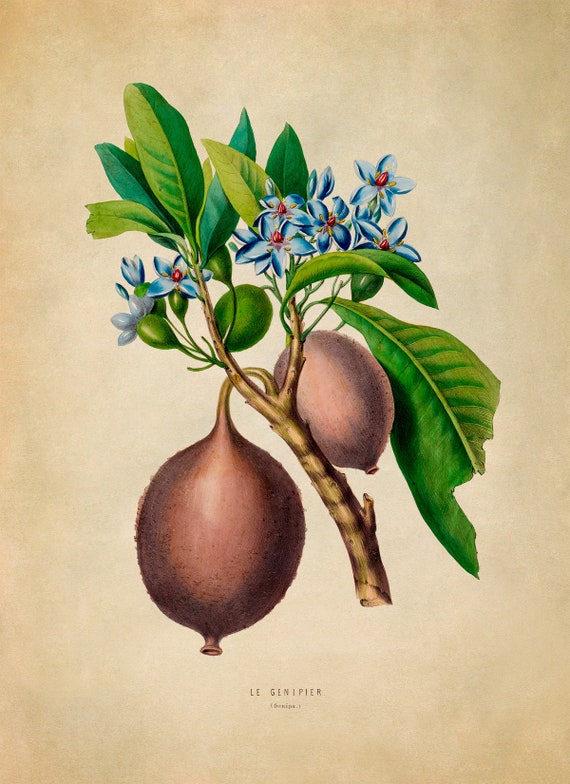This is a detailed color illustration drawn with colored pencils on weathered white paper, exhibiting a background with a faded beige hue. The image showcases a branch that tilts to the left, adorned with numerous vivid green leaves and light blue flowers, likely jasmine, which have white centers tinged with red. Along this branch, two apricot-like fruits are suspended; the larger, more mature fruit, rich in brown hues, hangs heavily and sags from the branch, while the smaller, lemon-sized fruit appears less ripe and less brown. The leaf at the far right of the branch is notably ripped at the bottom. At the very bottom of the image, the text "LE GENIPIER" is written, with "GENIPA" in parentheses beneath it. The illustration possesses an elegant quality, featuring a sophisticated color scheme of reds, greens, and blues, with a touch of beige in the background.